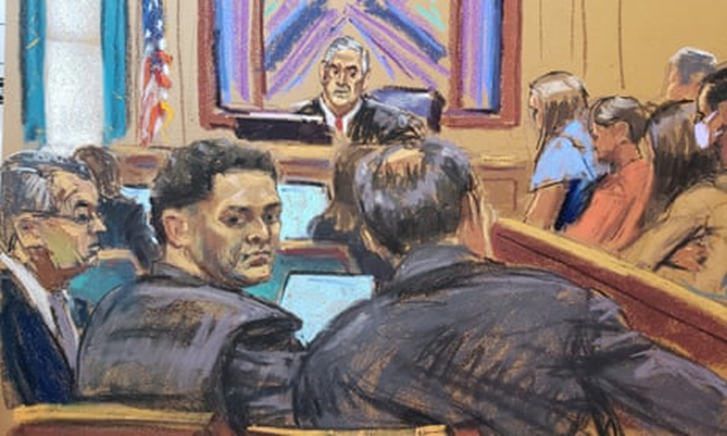The artwork, rendered in the style of a court reporter's drawing, presents a detailed courtroom scene. At the center, a white-haired judge is depicted wearing a black robe, a tie, and is seated behind a black screen with an American flag to his left. Behind the judge, a painting in blue, purple, and tan colors, framed in brown, hangs on a beige wall. The background features more beige tones and blue curtains that frame the scene.

In the foreground, there is a diverse group of individuals in formal attire, indicative of a courthouse setting. To the judge's right, a man with curly black hair and a darker complexion, wearing a suit, looks back towards the viewer with a concerned expression. Next to him, a white man with glasses in a blue suit sits composed. Further left, another man, viewed from behind, is partially balding with dark hair, also dressed in a suit.

On the right side, jury members or spectators are seated on the courtroom bench. Among them, a man wearing a face mask and a woman in an orange shirt are notable. Another woman in blue sits beside them. The courtroom scene is further accented by multiple computer screens positioned in front of the individuals, enhancing the modernity of the setting. The judge appears to be overseeing the proceedings attentively, adding a sense of gravity to the depicted moment.